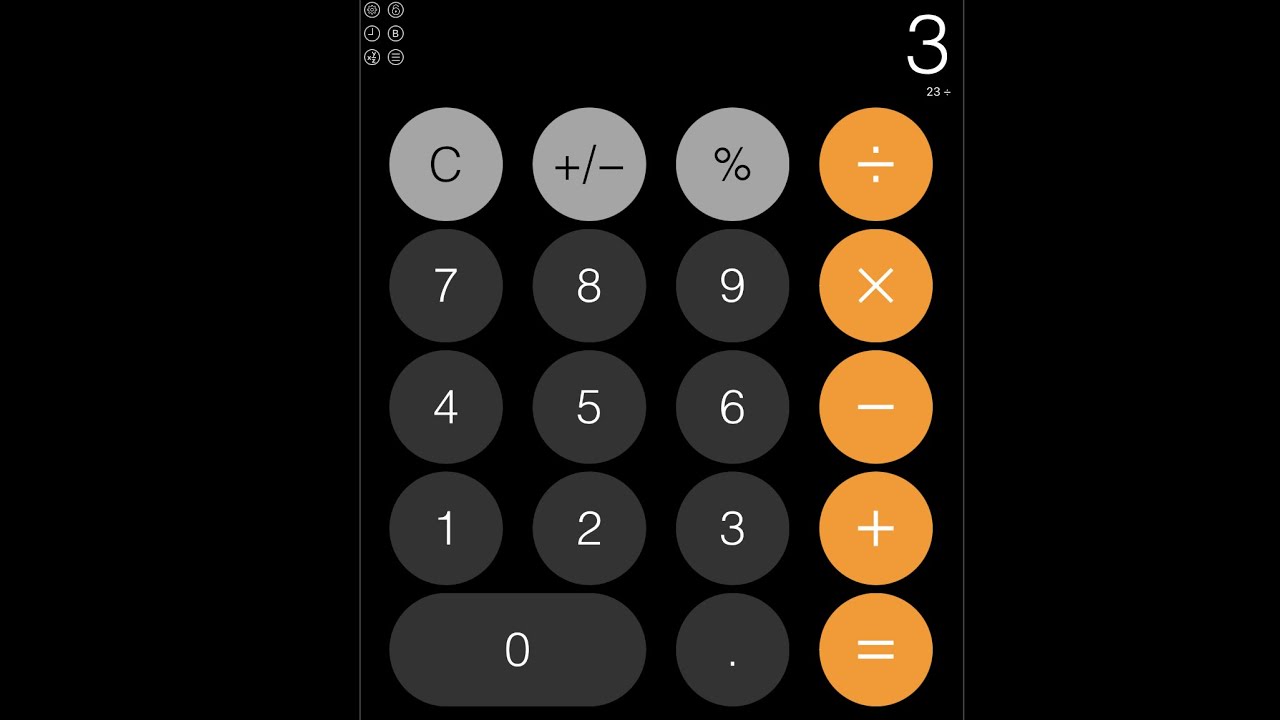This is a detailed screenshot of a calculator app set against a black background. At the top right corner of the screen, the number "3" is displayed in white. The calculator interface below this number is organized into a grid of buttons, structured as follows:

- **Top Row:** Gray button with "C" for clear, gray button with a plus/minus symbol, gray button with a percent symbol, orange button for division.
- **Second Row:** Dark gray buttons for the numbers 7, 8, and 9, followed by an orange button for multiplication (X).
- **Third Row:** Dark gray buttons for the numbers 4, 5, and 6, followed by an orange button for subtraction (minus).
- **Fourth Row:** Dark gray buttons for the numbers 1, 2, and 3, followed by an orange button for addition (plus sign).
- **Bottom Row:** A dark gray button for the number 0, a dark gray button for the decimal point, and an orange button for the equal sign.

This image strictly features numeric and operational symbols typical of a digital calculator interface. It contains no photographic elements, including people, animals, or plants.